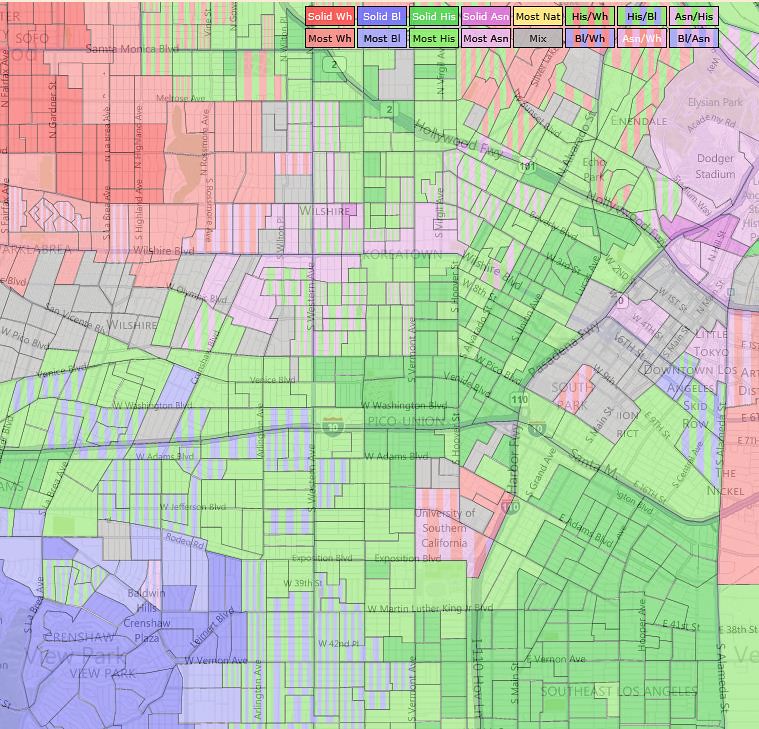The image showcases a detailed map, presumably of a city, occupying the entirety of the photograph. The upper right quadrant of the map features a legend organized into two rows, comprising a total of 16 squares, with eight squares in the top row and eight in the bottom. Each square in the legend explains the meaning of the various colors that segment the map, which appear to denote different property lines or zones within the city. Key locations such as "South Park" and the "University of Southern California" are notably labeled. Additionally, the map includes symbols indicative of routes and highways, providing further context and navigational aid.